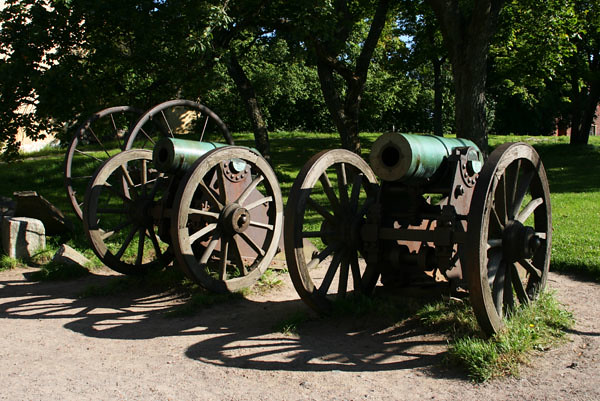The photograph captures an outdoor, park-like setting featuring at least two old-fashioned cannons as the focal point. These cannons are situated on a dirt and sandy area with patches of grass growing around and beneath the wheels. The cannons themselves have green barrels and large wheels, which are brown and appear to have wooden centers with metal framing. Behind the cannons, there is a well-maintained, green lawn leading to a backdrop of numerous full, leafy trees with dark trunks. The trees cast significant shadows on the ground, revealing limited sunlight permeating through their dense foliage, though sunny patches of grass are also visible. The scene is complemented by a blue sky peeking through the treetops and a tan building to the left. In the foreground, the cannons are depicted with their barrels aimed outward, ready to fire, and you can notice shadows cast by the cannons on the ground, adding to the historical ambiance of the image.